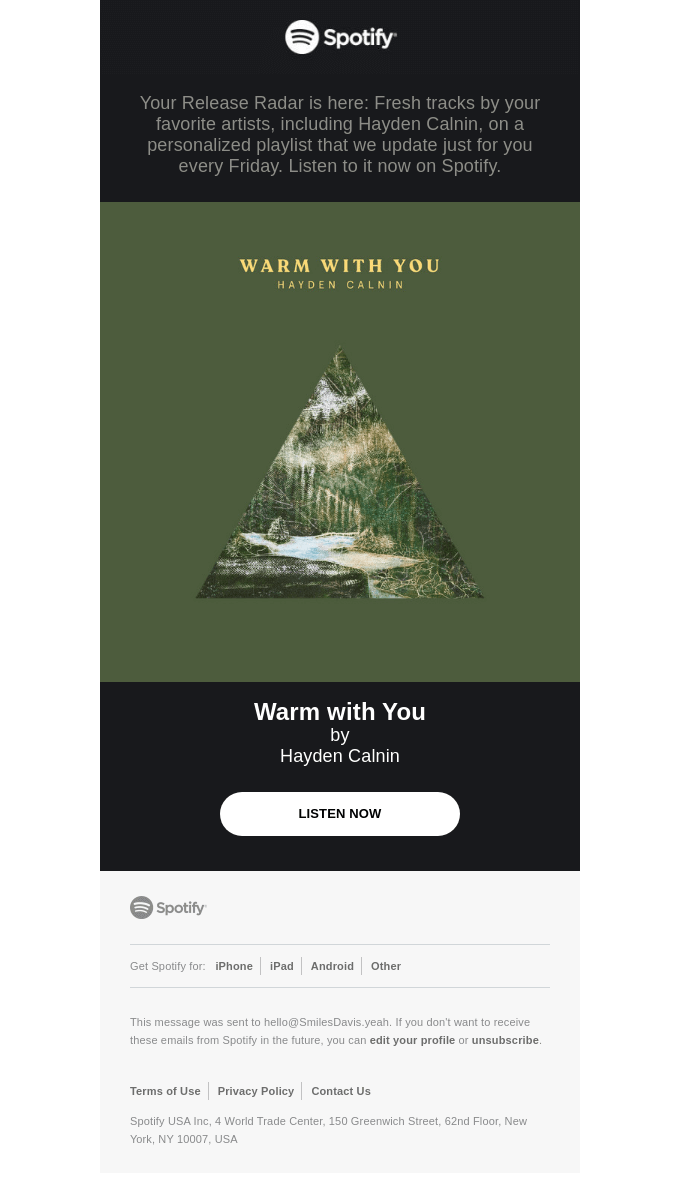A miniature Spotify advertisement screenshot features a clear identification through its prominent white Spotify logo at the top, paired intricately with a white circle and black soundwave icon. The ad headline in gray text announces, "Your Release Radar is here," highlighting the arrival of fresh tracks by favorite artists, such as Hayden Khan, on a personalized playlist updated every Friday. The mid-section displays an artistic cover with the title "Warm With You" by Hayden Cullen, set against a whimsical, forested scene resembling a sunset painting. Completing the layout, the bottom of the ad reiterates the song "Warm With You" by Hayden Cullen and features a prominent white "Listen Now" button with black text, inviting immediate engagement.